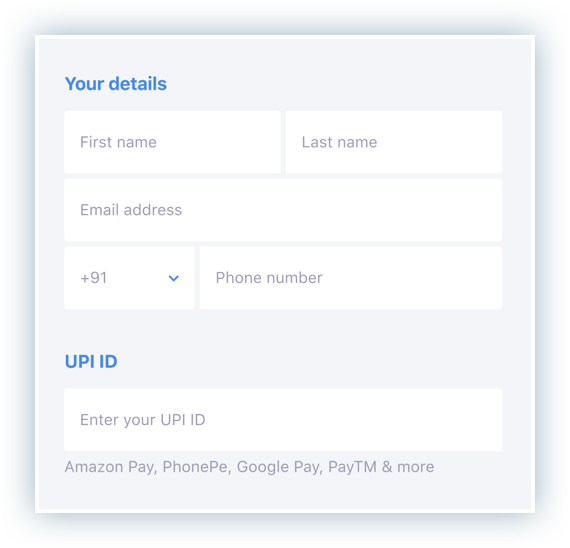The image is a square screenshot displaying a webpage that is requesting personal information. The image itself is bordered by a dark gray, faded shadow effect and is outlined in white. The interior of the square is filled with a gray background. 

In the upper left-hand corner, blue text reads "Your Details." Below this, there is a vertically arranged section for user entry fields. The first line contains two horizontal boxes: the left box is designated for the user's first name and the right box for their last name. 

Beneath these name fields, there is a long, horizontally placed rectangular box with a white background labeled for the user's email address.

Further down, there are fields for phone information. On the left, a smaller box shows the country or area code defaulted to "+91". To the right of this, there is another box intended for the user's phone number. There is a noticeable blank space, offering visual separation between sections.

Towards the bottom left, blue text reads "UPI ID" accompanied by another long rectangular box where users can enter their UPI ID. Underneath this, text indicates supported digital payment options: "Amazon Pay, PhonePe, Google Pay, PayTM, and more."